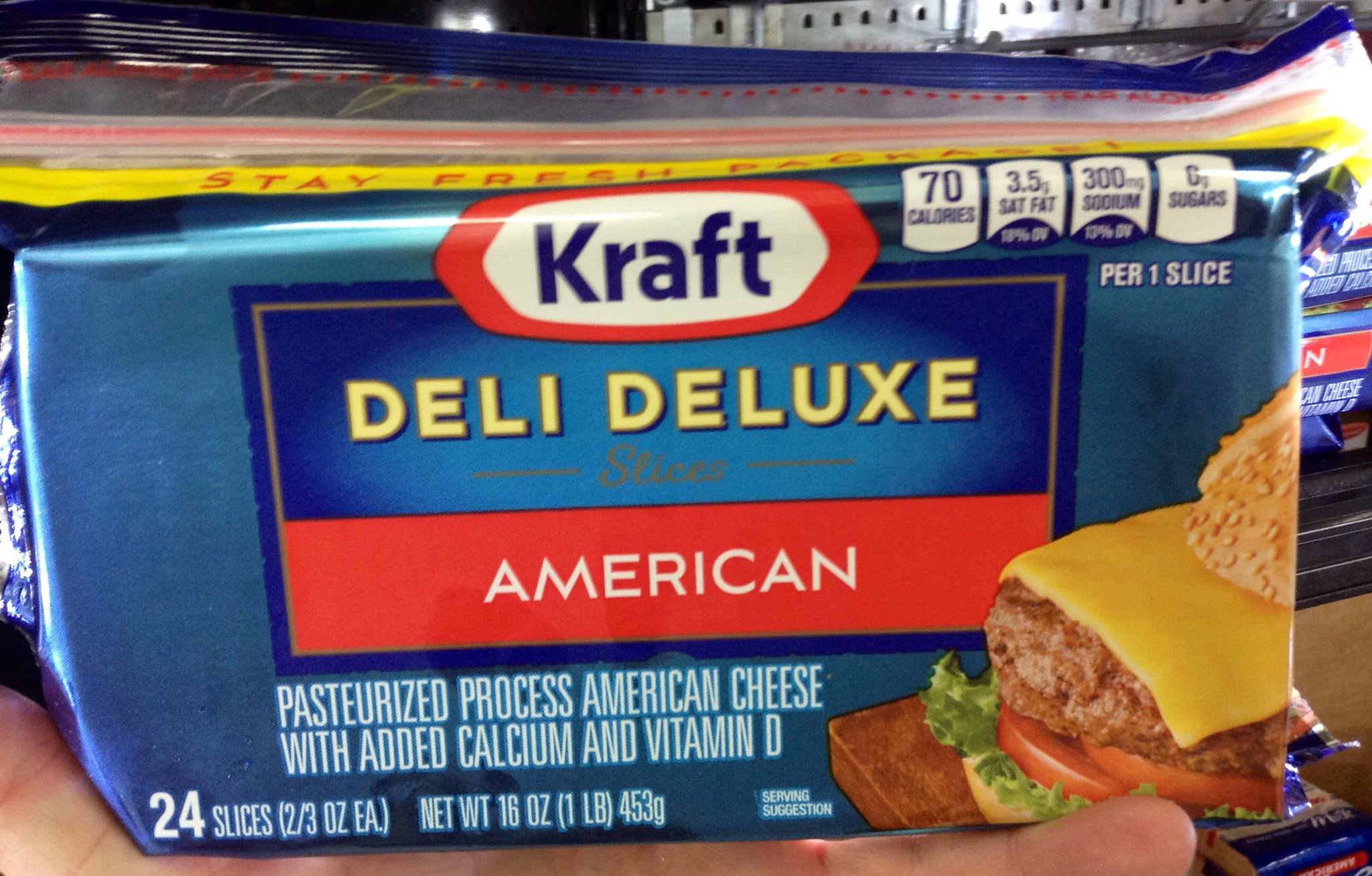This is a close-up photograph of a package of Kraft Deli Deluxe American Cheese Slices. At the top of the package, the iconic Kraft logo is prominently displayed, featuring blue text on a white background with a red backdrop behind the white field, ensuring high visibility. Below the logo, "Deli Deluxe" is inscribed in crisp white text, which is followed by the word "Slices" in a soft gray hue. The term "American" is clearly written in white text beneath these labels. On the right side of the packaging, a tantalizing image of a freshly made hamburger is showcased, complete with vibrant red tomatoes, crisp green lettuce, and a rich slice of American cheese, all nestled within a sesame seed bun. The overall color scheme of the package is primarily a deep blue, making the vibrant colors and text stand out effectively.